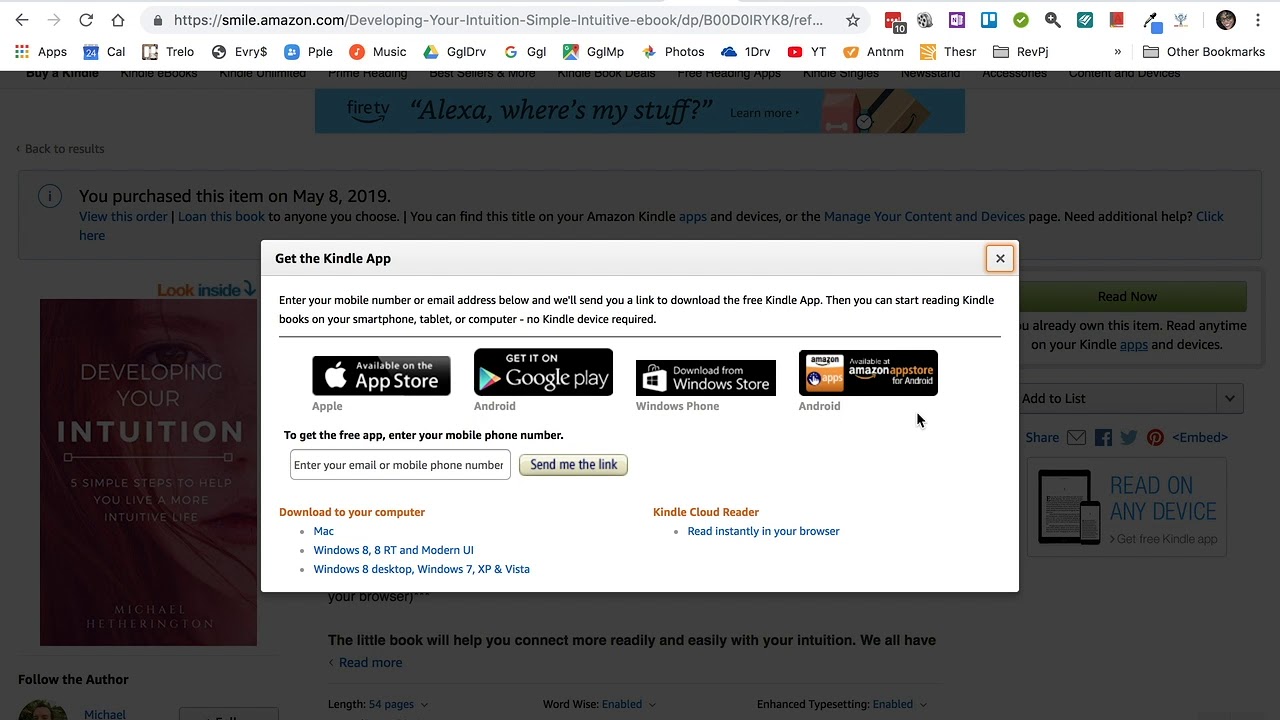A screen capture from a desktop computer showcases the website https://smile.amazon.com, as indicated by the web address in the white horizontal bar at the top. The main body of the image is slightly grayed out, revealing a dimmed background beneath which features a blue horizontal bar displaying the text, "Alexa, where's my stuff?" Central to the image is an open window with a white background. At the top left corner of this window, the text reads, "Get the Kindle app." Below this header, in fine print, instructions state, "Enter your mobile number or email address below and we'll send you a link to download the free Kindle app. Then you can start reading Kindle books on your smartphone, tablet, or computer. No Kindle device required."